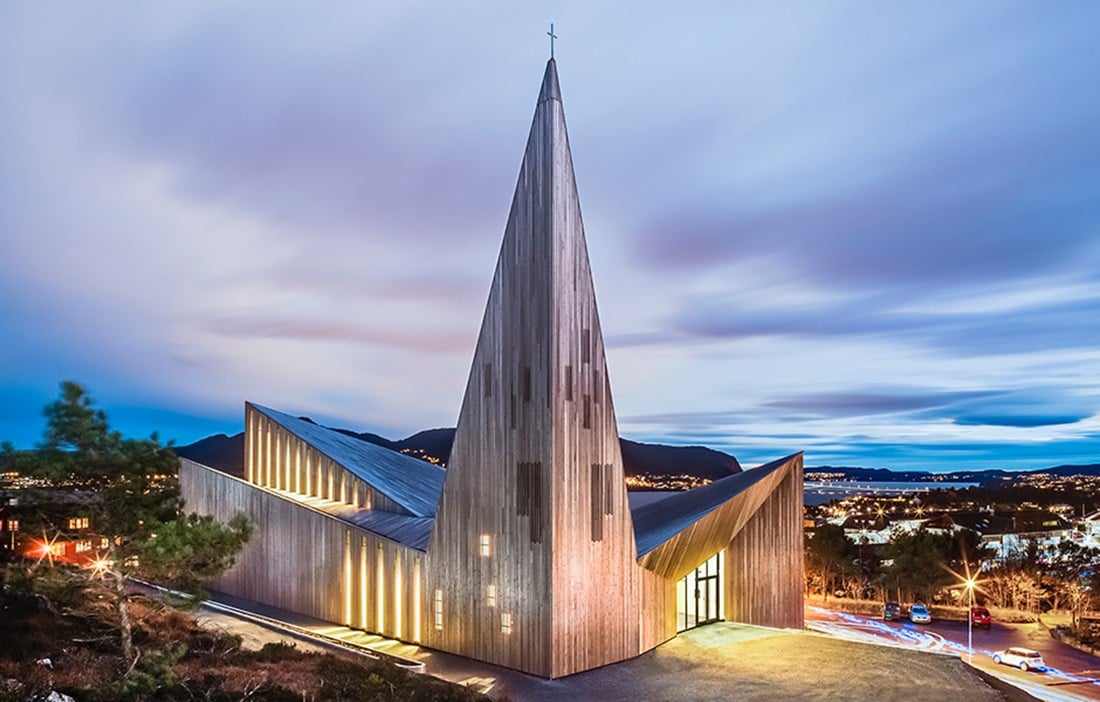The image depicts an ultra-modern, cathedral-like church situated atop a hill at dusk. The architecture is strikingly contemporary, featuring a central isosceles triangular structure that soars 100 to 200 feet high, crowned with a small cross. Flanking this centerpiece are various trapezoidal elements and jutting triangular sections, creating a dynamic and angular design. The exterior is a mix of dark gray and silvery hues, with wooden paneling accentuating the edges. 

Large, floor-to-ceiling rectangular windows are illuminated from within, highlighting the lower parts of the central triangle, while additional, darker windows punctuate higher sections. A prominent trapezoid-shaped entrance with double glass doors and a wooden overhang is visible, inviting visitors inside. 

In the background, a cityscape adorned with twinkling lights stretches towards a body of water, likely a lake, as suggested by the thin sliver of blue. The sky, transitioning from blue to darker shades with hints of pink and white clouds, enhances the serene twilight ambiance. The church overlooks this urban landscape, with faint signs of a street and a few cars visible near its base, completing this tranquil yet striking scene.